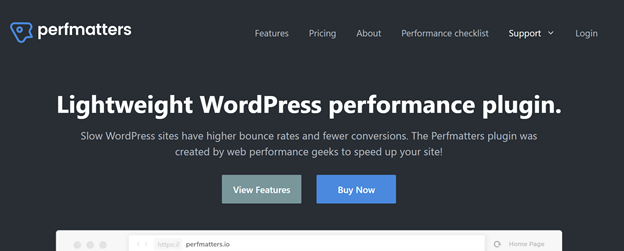Cropped screenshot of the Perfmatters website, showcasing its dark-themed interface with a soft black background. The highlighted text announces "Lightweight WordPress Performance Plugin" and emphasizes that "Slow WordPress sites have higher bounce rates and fewer conversions." The Perfmatters plugin, developed by web performance experts, aims to optimize site speed. Users are prompted with options to "View Features" or "Buy Now." The top navigation menu includes sections for Features, Pricing, About, Performance Checklist, Support, and Login. Part of a browser window displaying perfmatters.io is visible at the bottom, indicating a possible cut-off image of the site. The intention behind using the plugin is not only to enhance performance but also to improve business metrics like clicks and conversions. Next to the Perfmatters text, there's a minimalist logo resembling a spaceship.